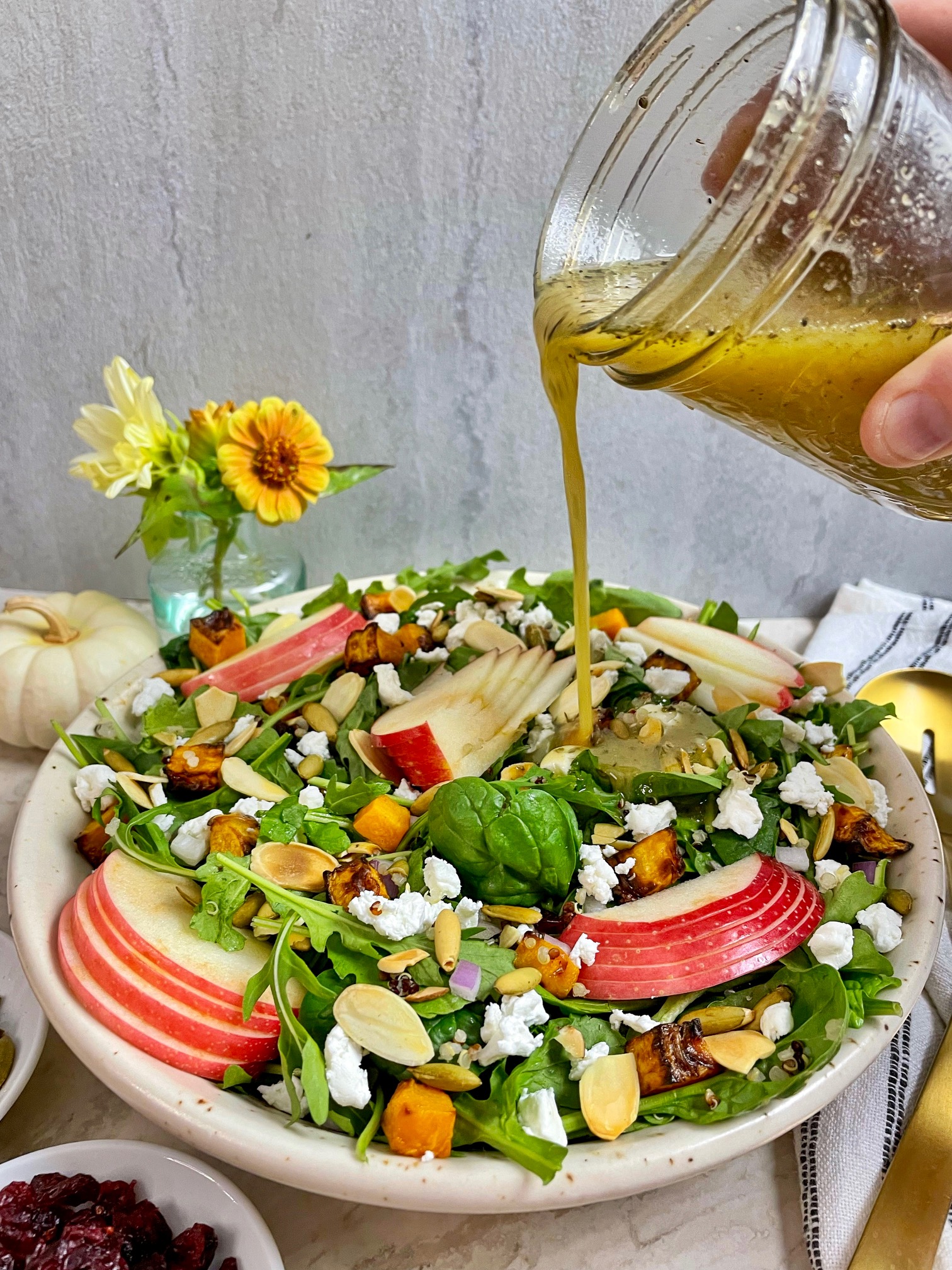In the image, there's a round white plate brimming with a vibrant salad. The plate rests on a table adorned with a tablecloth, a small potted plant, a white pumpkin, and a couple of bowls situated on the bottom left. A spoon lies nearby, ready to serve. The salad itself is a colorful mix featuring sliced red apples, fresh green leaves, slivers of almonds, and bits and pieces of cottage cheese. There are also striking yellow and black elements scattered throughout, adding to the visual appeal. At the top right corner of the image, a hand is seen pouring a jar of yellow vinaigrette dressing onto the salad, enhancing its flavor with a final touch.